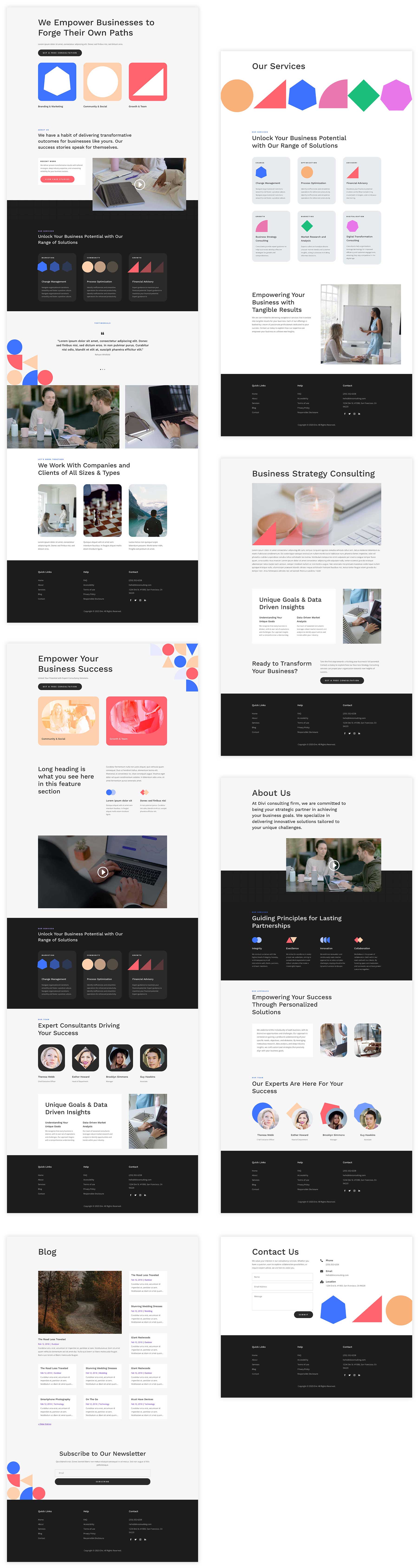The image features a vertically elongated frame displaying two side-by-side screenshots of a web page or mobile app. The vertical orientation of the screenshots, combined with the narrow framing, makes it challenging to discern specific textual content. However, the layout exhibits a sequence of sections, each delineated by a black horizontal banner. Interspersed throughout the sections are various geometric shapes in bright colors, including orange, red, blue, pink, green, and purple, lending a vibrant and dynamic quality to the overall design. Additionally, several areas contain photo-like images, although their content remains indistinguishable. The arrangement and repetition suggest that the image may consist of multiple stacked and spliced-together screenshots from different parts of the same website or app interface.